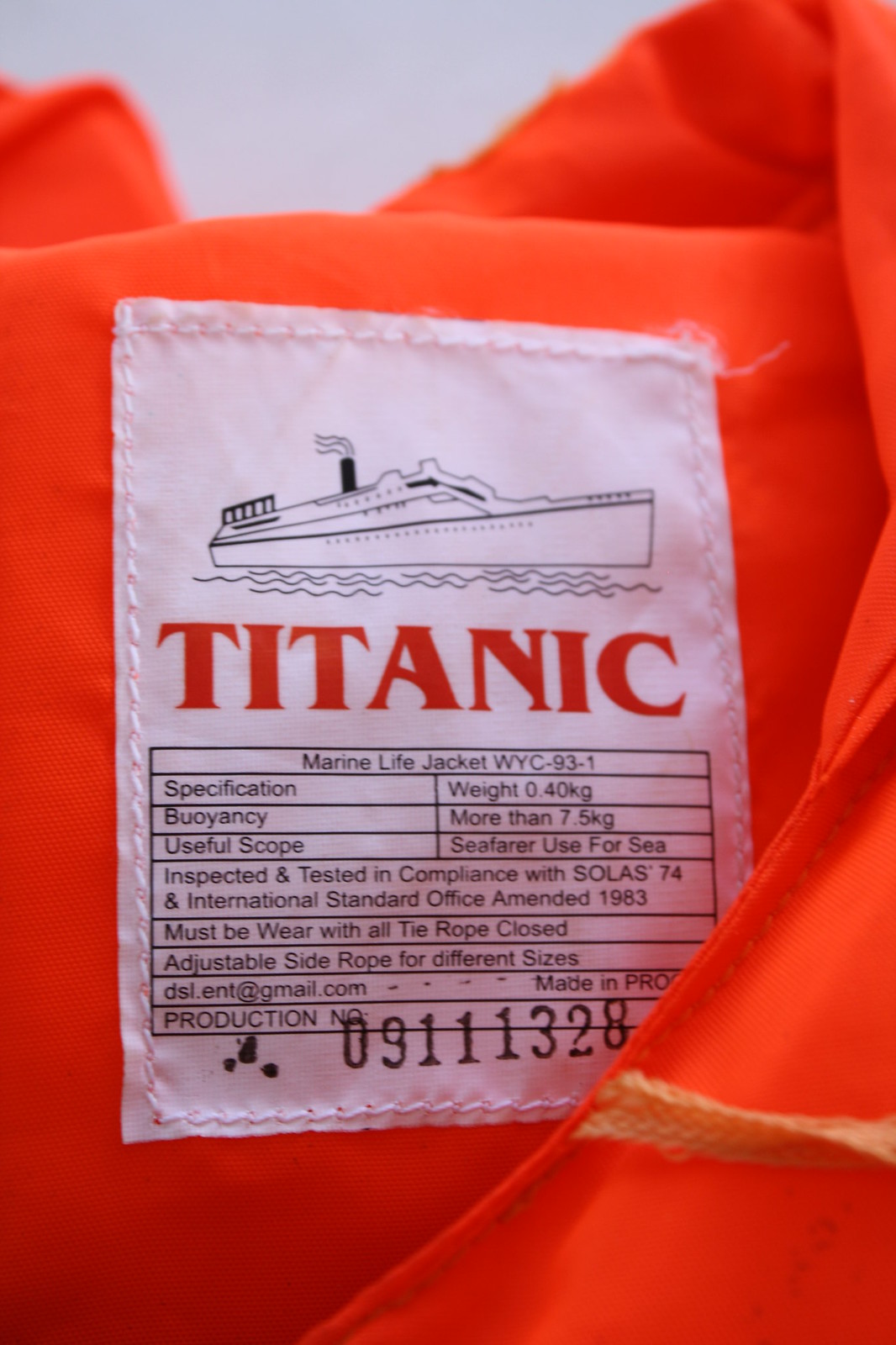**Detailed Caption:**

In this image, we see the interior tag of a bright orange piece of clothing, specifically a marine life jacket. The tag features a drawing of a large luxury ship with a smoke stack, sailing on water, likely symbolizing the life jacket's maritime purpose. The text "Titanic" is prominently displayed in orange, evoking the infamous ocean liner. The tag includes detailed specifications: model WYC 93-1, weight 0.40 kg, and buoyancy of over 7.5 kg. It states the item is intended for seafaring use, with a useful scope marked as "4C." Compliance information indicates the life jacket has been inspected and tested in accordance with SOLUS 74 and the amended International Standard Office regulations from 1983. Instructions mention the need to wear the life jacket with all tie ropes securely fastened and note that adjustable side ropes can accommodate different sizes. A visible red string, which is actually orange, protrudes from the fabric, adding a final touch to the detailed view of this essential safety equipment.